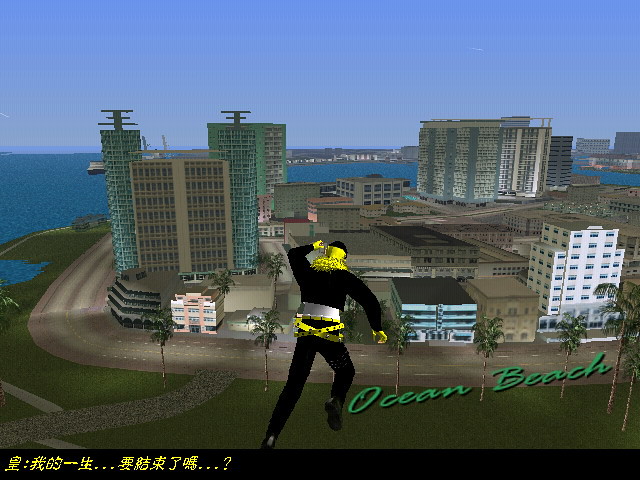The image is a colorful computer-generated screenshot from a game, with the words "Ocean Beach" diagonally at the bottom right corner and some text in an Asian alphabet at the bottom left. The central focus is an avatar dressed in black with yellow accessories, including gloves, a belt, and a ruffled collar, appearing to jump off a mountain or building towards Ocean Beach City. The urban landscape features a mix of taller condos and apartment buildings, along with shorter businesses, hotels, and motels, all set against the backdrop of a wide highway that wraps around the town area. Beyond the dense arrangement of buildings lies a bay, leading to another section of the city. The scene is completed with palm trees to the right and a stretch of grass and walking paths, all under a blue sky. Construction cranes are visible in the distance, indicating ongoing development. The water in the background deepens the scenic view.